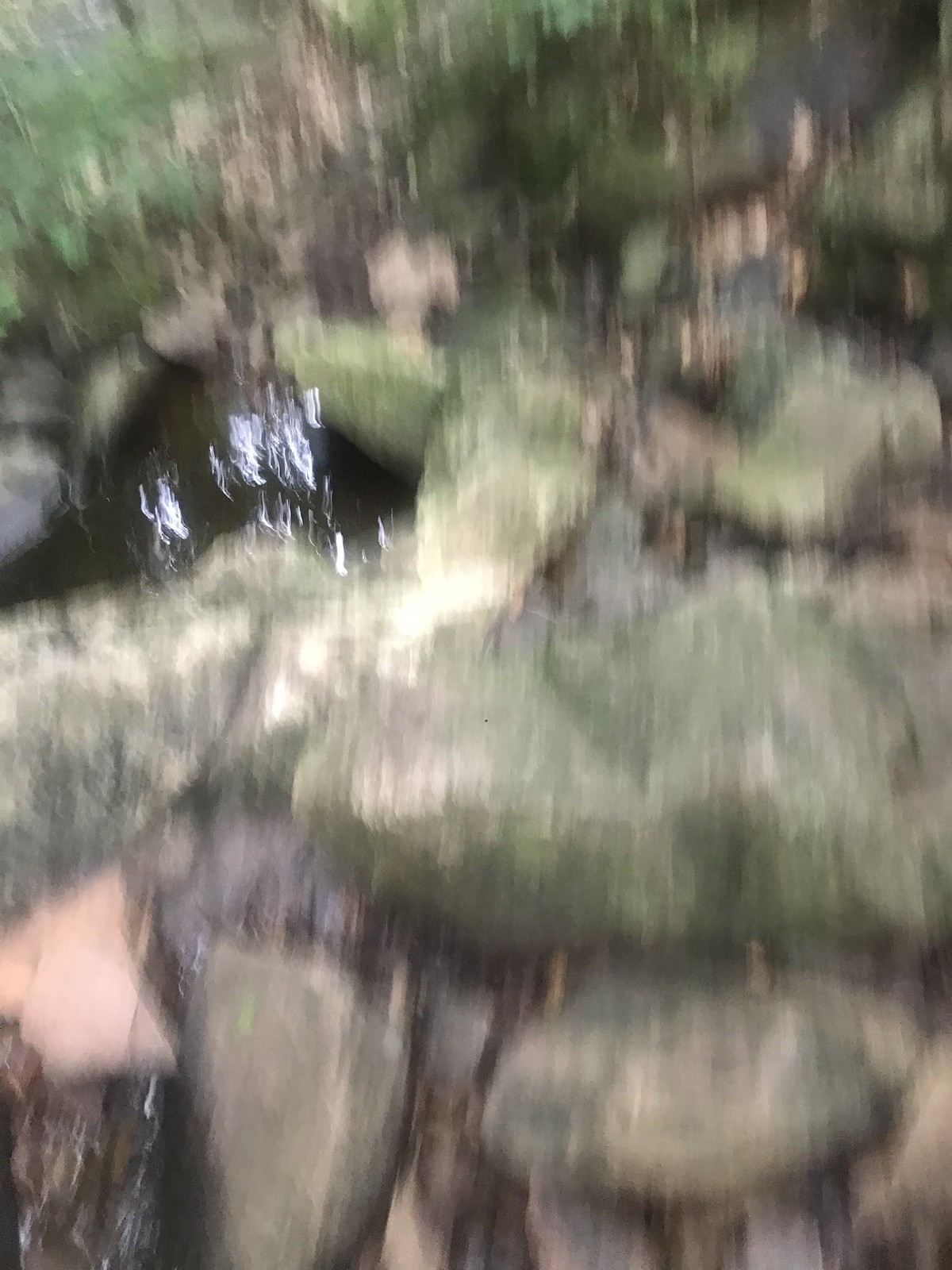The image depicts a heavily blurred outdoor scene, giving the impression of being hastily captured while in motion, possibly as the photographer moved quickly through a forest. The dominant colors are green, grey, and beige, with multiple vertical streaks adding to the overall blur. In the foreground and midground, large, indistinguishable boulders and rock formations are present. To the left side of the image, there seems to be running water, forming what looks like a creek surrounded by rocks. The background reveals hints of greenery from bushes or trees, blending with the rugged terrain of rocks and leaves scattered on the ground. Adding a sense of curiosity, a blurry, brownish animal appears to be emerging from a small cave or hole amidst the rocks. Overall, the scene combines elements of forest floor debris, water, and dense vegetation, all heavily obscured by motion and blur.